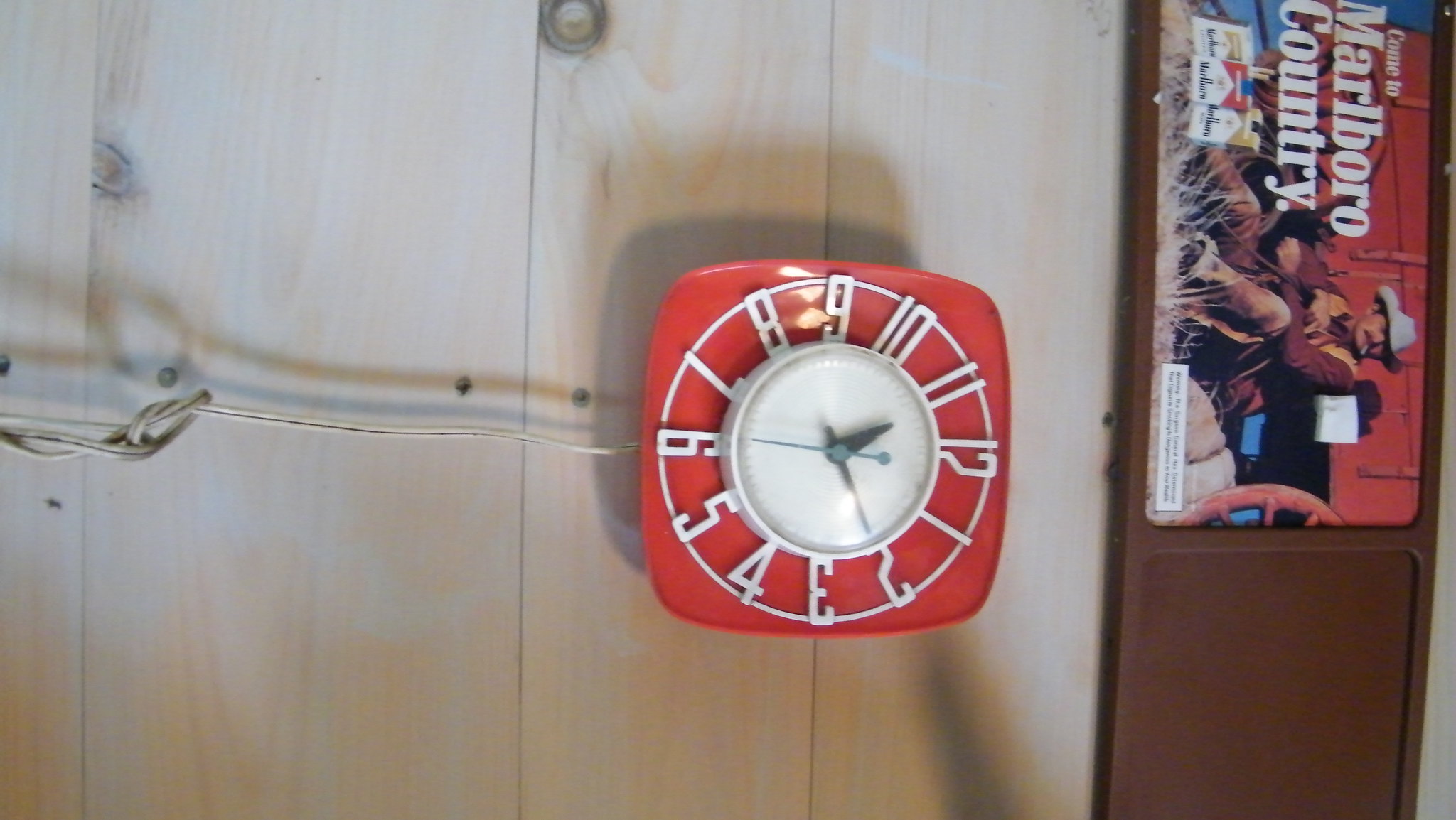This photograph, rotated 90 degrees, features a wall-mounted clock. Positioned to occupy approximately 20% of the central frame, the clock appears to extend sideways due to the image's tilt, giving the illusion that its power cord, emerging from its bottom, stretches out from the left side. The clock’s casing is strikingly red, adorned with silver numbers arranged in a circular pattern. At the heart of its design is a white dome that houses the clock's movement hands. The hands are distinctly colored, with a black hour hand, a black minute hand, and a blue second hand, providing a subtle yet notable contrast against the white background.